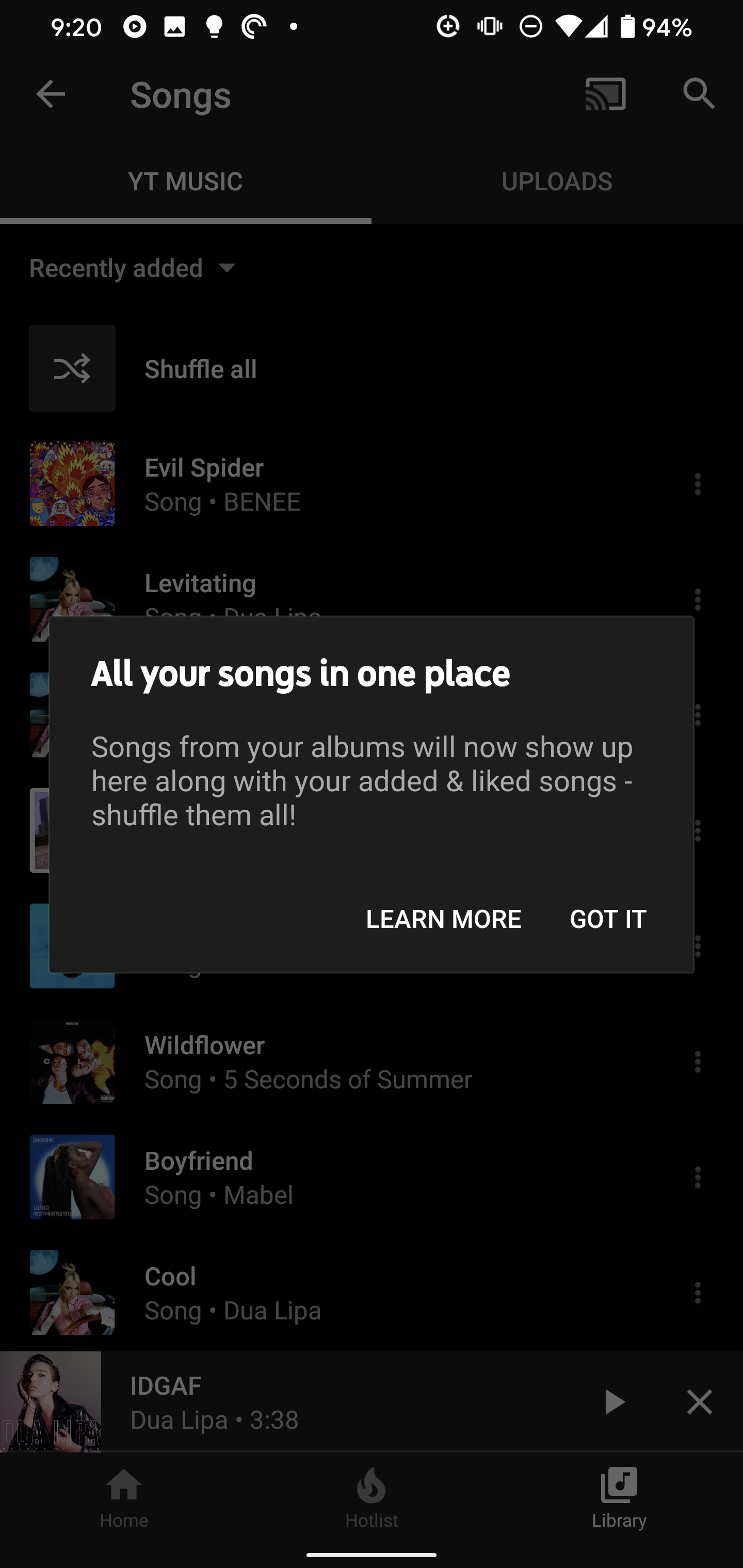The image showcases a music app interface opened on a mobile phone. The time displayed at the top of the screen is 9:20. At the very top, the screen features several icons, including a play button, a light bulb, and a photo icon. In the upper right corner, there are additional icons for adding a new item (plus sign), do not disturb mode, vibrate mode, Wi-Fi, data connection, and a battery level indicator showing 94%.

Below these icons, a gray box with a message pops up, informing the user that all their songs are now consolidated in one place. The message reads: "All your songs in one place. Songs from all your albums will now show up here along with your added and liked songs. Shuffle them all. Learn more. Got it."

Behind the message, the interface of the app is slightly grayed out but still visible. The app features several categories and listings. It says "Songs" at the top, accompanied by a Chromecast-style logo. Below this, the app lists "YT Music" and "Uploads" categories. Additionally, there is a "Recently added" section with options to shuffle all songs. Songs listed include "Evil Spider" by Bene, "Levitating" by Dua Lipa, "Wildflower" by 5 Seconds of Summer, "Boyfriend" by Mabel, "Cool" by Dua Lipa, and "IDGAF" by Dua Lipa. The time stamp at the bottom right of the song list reads 3:38.

At the bottom of the screen, there are three selectable options: "Home," "Hotlist," and "Library."